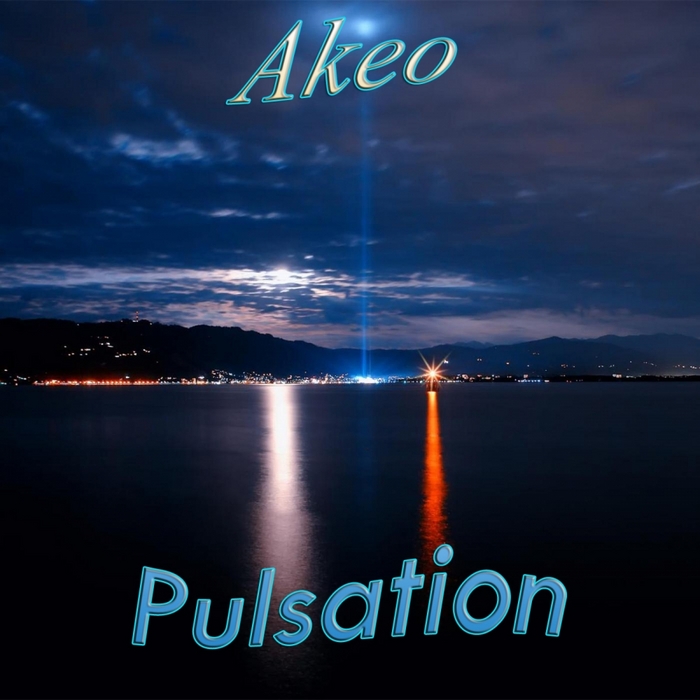The image captures a tranquil bay at sunset, framed by a mountainous shoreline dotted with city lights and coastal establishments. The foreground is dominated by the calm and reflective waters of the bay. On the shore, two prominent lights stand out—one white and the other orange—casting their shimmering reflections on the water. Between these lights, a striking blue light, seemingly from the sky, pierces down, adding an ethereal touch to the scene. The sky itself is heavily clouded, allowing minimal sunlight to filter through, casting a dusky, moody ambiance over the entire setting. The words 'ECHO' are inscribed in bold blue letters at the top center of the image, while 'PULSATION,' also in blue, is prominently displayed at the bottom center. The distant hills roll gently toward the bustling town, enriching the skyline with their natural contours.